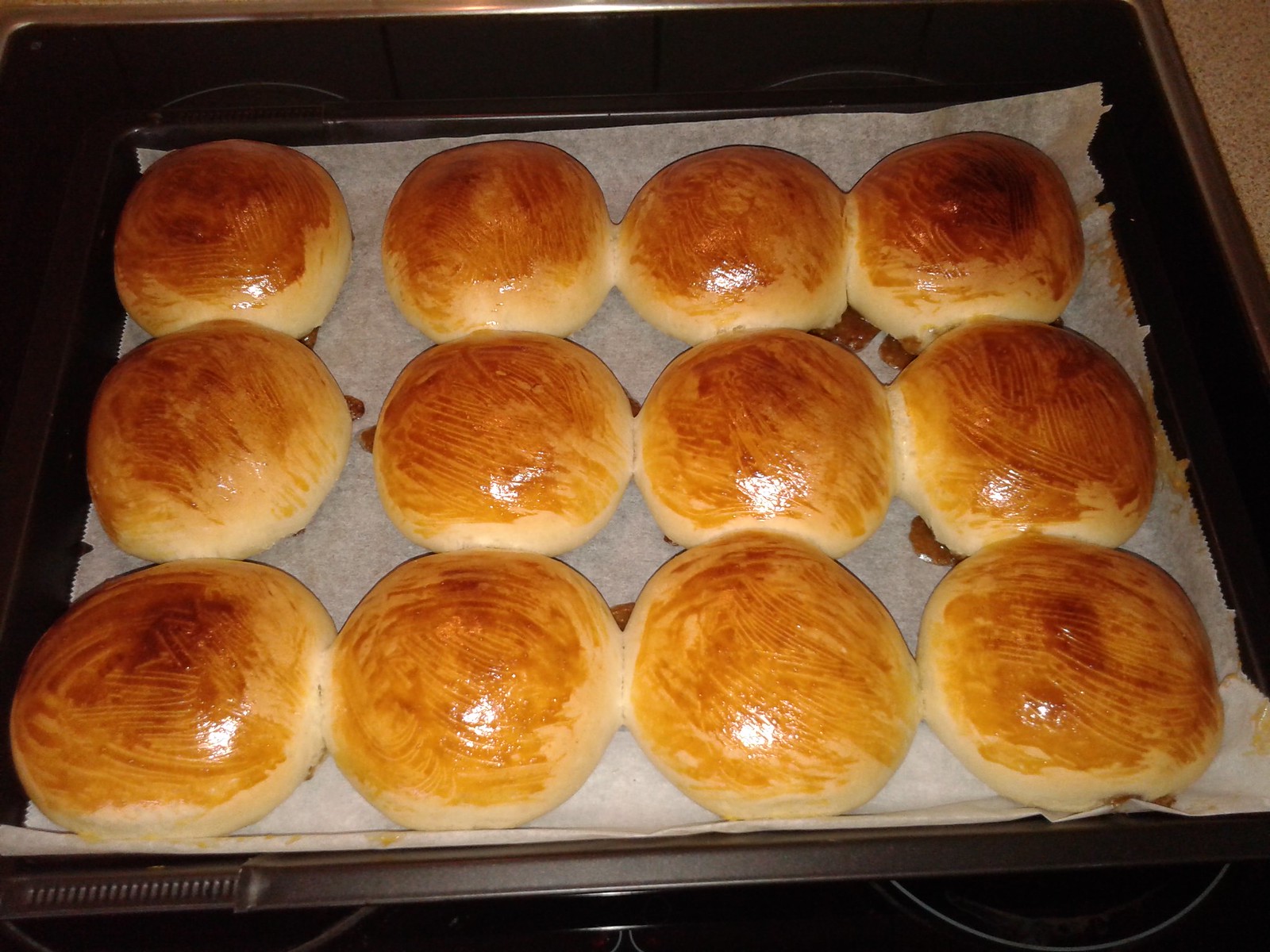The image captures a rectangular silver pan lined with white parchment paper, holding freshly baked, glossy dinner rolls that are perfectly arranged in three rows of four. The rolls are plump and round, starting with a light beige hue at the bottom and transitioning to a rich dark brown on top, indicating a delightful buttery finish. They appear to have just come out of the oven or are about to go in, exuding an inviting warmth and a delectable aroma reminiscent of Thanksgiving Day treats. The pan sits on a stovetop, with the silver curves of a burner and a medium brown countertop visible in parts of the background. The rolls are closely nestled next to each other, their shiny surface hinting at an egg wash or butter glaze, enhancing their appetizing look.